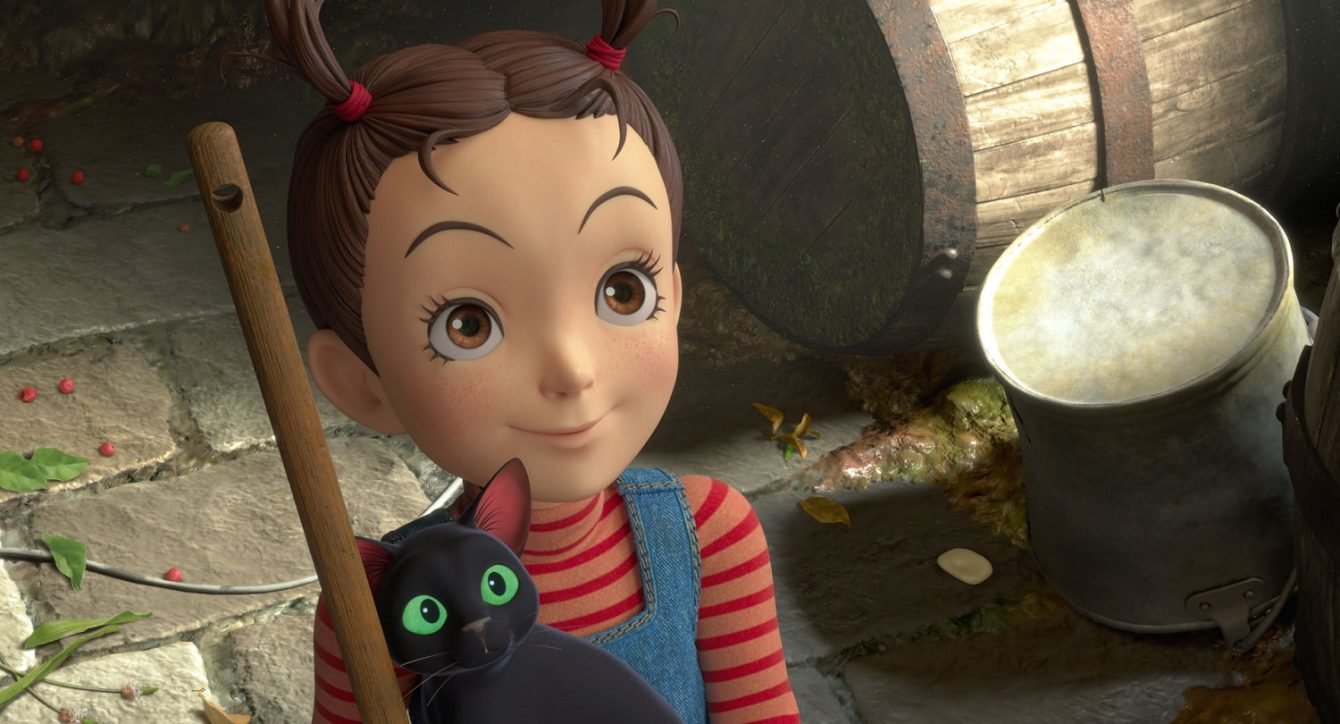The CGI image portrays a young girl depicted in an animated or cartoon style, holding a black cat prominently near her chest. The girl, positioned centrally to the left, has wide hazel eyes that gaze upwards to the right with a surprised yet smiling expression. Her brunette hair is styled into two energetic pigtails that sprout vertically from her head, secured with red hair ties. She wears blue jean overalls over a long-sleeved shirt featuring light orange and red horizontal stripes. 

In her left hand, she clutches a vertical wooden-handled broom, standing upon a stone walkway. Surrounding her, the scene is dimly lit with shadows cast throughout, adding a moody ambiance. Red berries and green leaves scatter the ground, primarily concentrated to the left side. To the right, an overturned steel-gray bucket with a white interior and two barrels in various shades of rust and brown complete the background elements. The detailed setting behind the girl contributes to a rustic, somewhat mysterious atmosphere.